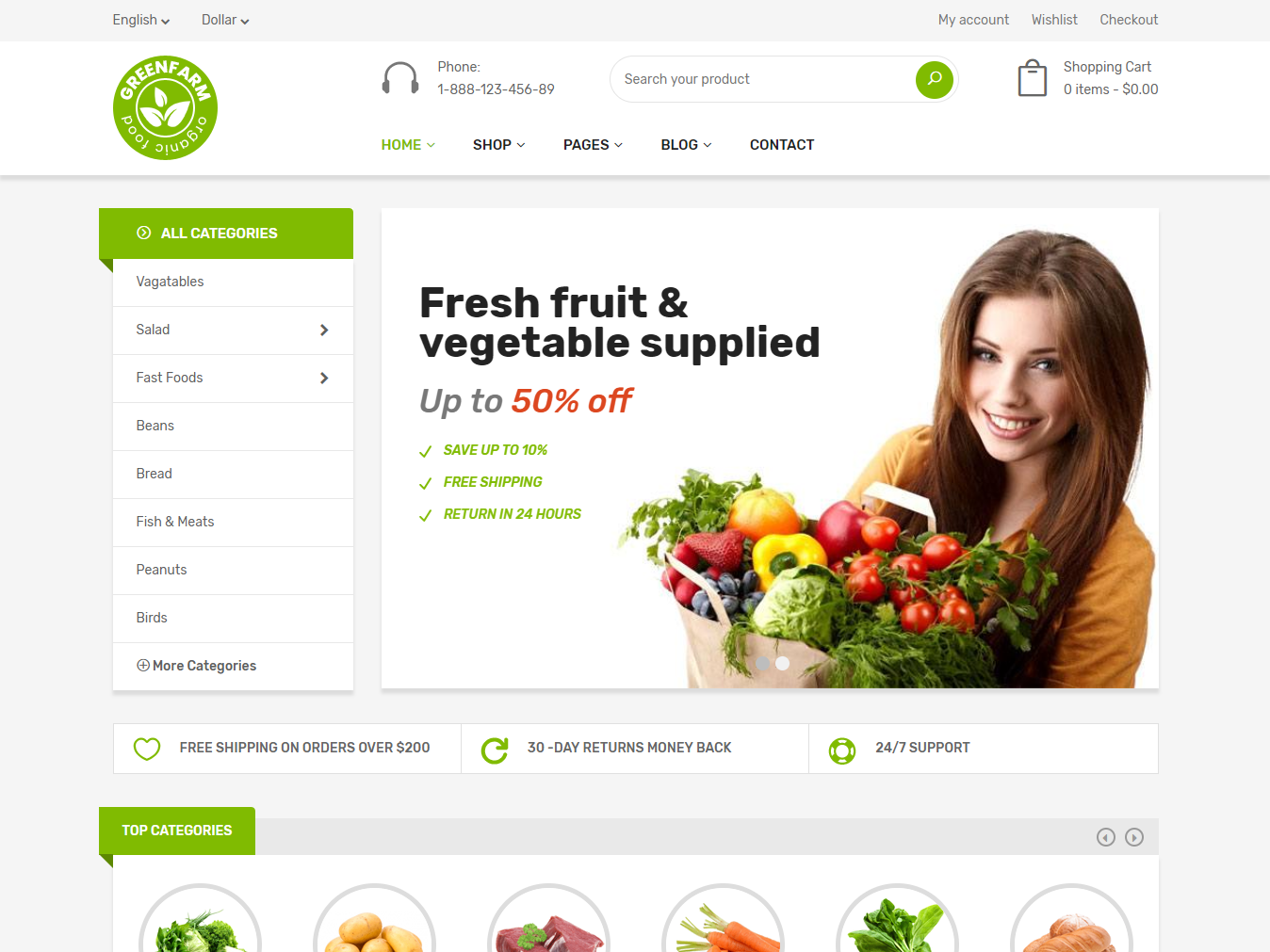At the top of the page, there's a gray bar featuring a language selector set to English and a currency selector configured to USD. On the right side of the bar, options for "My Account," "Wishlist," and "Checkout" are displayed. 

Below this, a white bar houses the website's logo, which consists of a green circle with a yellow ring and leaves inside, encircled by the words "Green Farms, Organic Food." A phone number is listed, alongside a search window, and an indication that the shopping cart is currently empty.

The main navigation menu below the white bar offers a drop-down list under "All Categories," enabling users to choose subcategories such as Vegetables, Salad, Fast Foods, Beans, Bread, Fish and Meats, Peanuts, Birds, and more. 

To the right of the navigation menu, there is a white box featuring a photo of a woman with long red hair wearing an orange top. She is holding a bag full of vegetables. The promotional text indicates that fresh fruit and vegetables are available at discounts up to 50% off, with free shipping and returns within 24 hours.

Proceeding further down, another white bar advertises "Free Shipping on Orders Over $200," "30-Day Returns," "Money Back Guarantee," and "24/7 Support."

In the green box below, labeled "Top Categories," there are gray circles containing images of various vegetables. Although some images are clipped, identifiable vegetables include potatoes, carrots, and greens, among others.